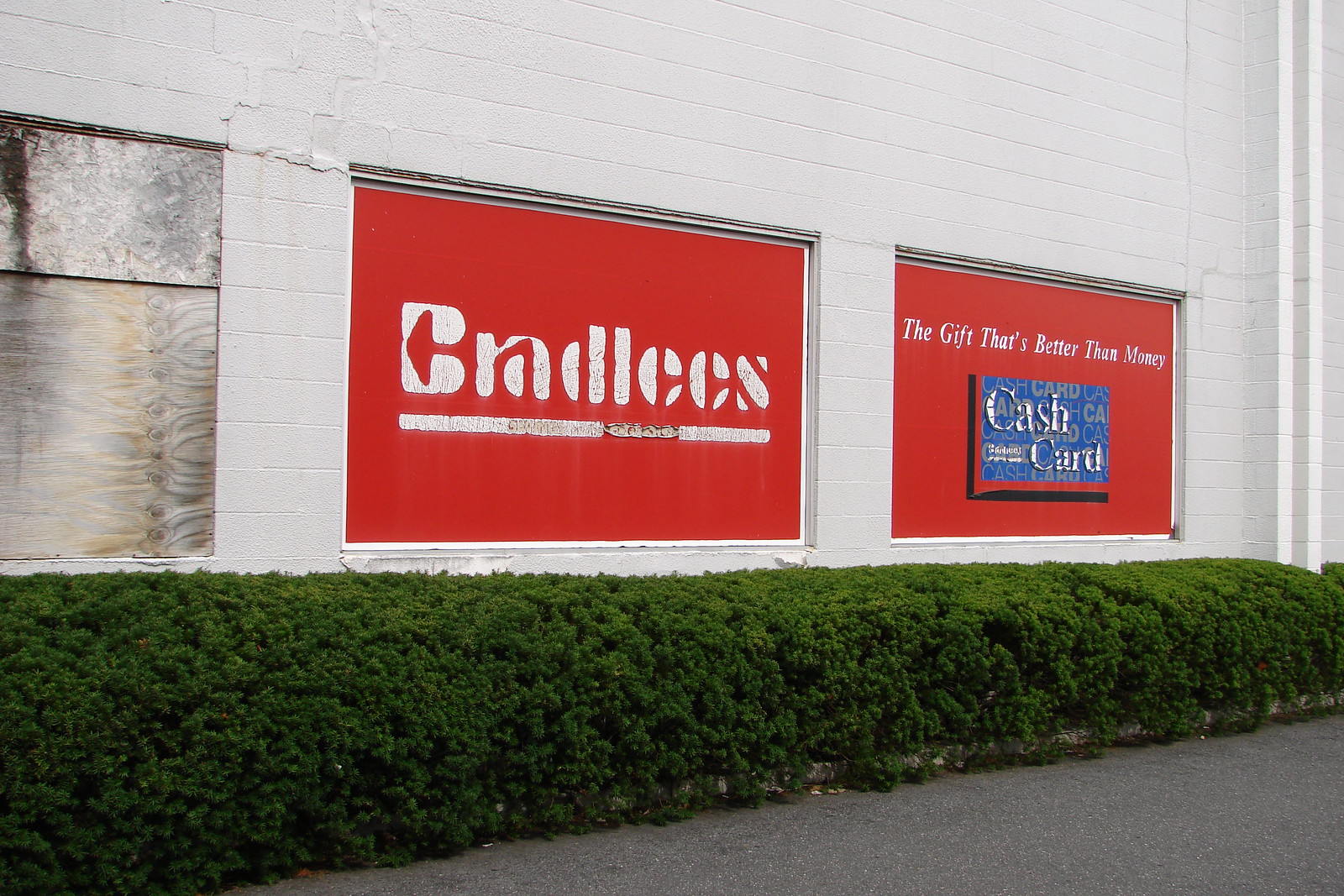In this horizontal photograph taken during the daytime, we see the exterior of a department store. The white cinder block building features a well-maintained row of green shrubs lining a gray concrete sidewalk that stretches diagonally from the lower right corner to the lower left corner of the image. Two prominent red signs stand out above the shrubs. The larger of the two signs, against a solid red background with white stencil-style lettering, reads "BRADLEY'S." To the right of this sign is another red sign with white print stating, "THE GIFT THAT'S BETTER THAN MONEY." Below this text, the sign features an image of a blue card labeled "CASH CARD." The blue card detail adds a touch of color contrast, drawing attention to the promotional message. The overall scene portrays a tidy and inviting commercial facade of Bradley's department store.